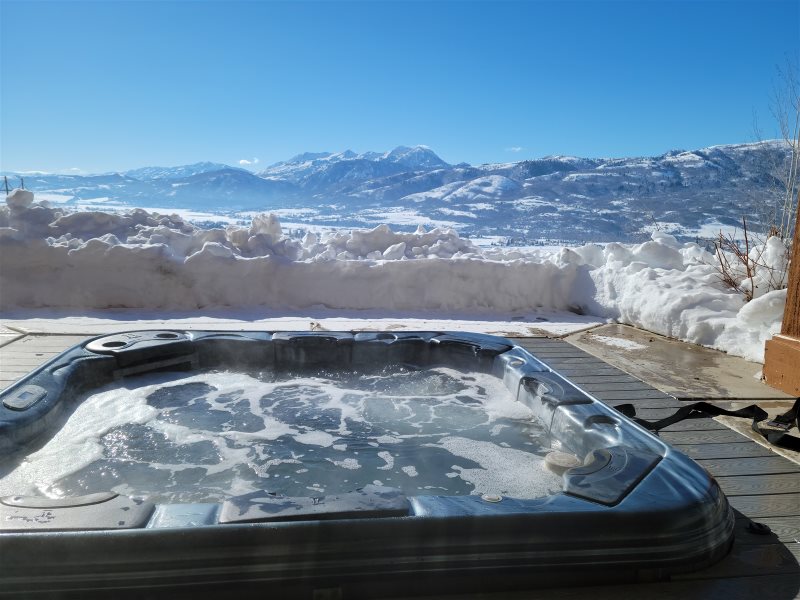The photo features a large blue and white marble hot tub, nestled on a gray wooden slat patio, positioned in the middle of a snow-covered landscape. Frost decorates the water's surface, and a gentle steam wafts off from the back of the hot tub, indicating it's turned on and bubbling. There's a notable clearing of packed snow around the hot tub, revealing the effort made to carve out access to this luxurious spot. The surrounding deck is bordered by what appears to be brown forts or potentially an ice fence, enhancing the cozy yet striking atmosphere. Towering in the background are majestic white mountains with a bluish tint, reflecting the clear, bright blue sky above. To the left, there might be a glimpse of a bridge blending into this winter wonderland scene.